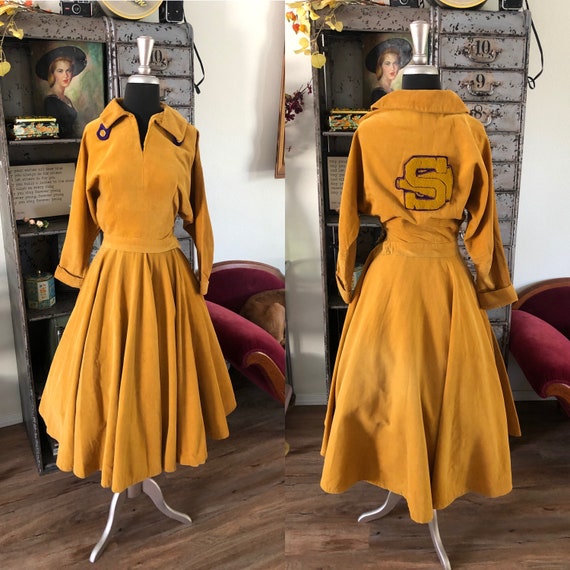The image consists of two photographs displayed side by side, showcasing the front and back views of a vintage school uniform dress, displayed on a headless mannequin. The dress is predominantly dark yellow (or orange) with long sleeves and cuffs, and it features a frilly skirt. In the background, a room with wooden flooring can be seen, containing various dated furniture items. Notably, there is a red chair and a portrait of a young lady with blonde hair, pink lipstick, and a black hat and dress. The room also includes labeled drawers (marked 10-9-8), shelves with assorted knickknacks, and other antique objects. The back of the dress features a large emblematic 'S' accompanied by a megaphone, elements commonly associated with cheerleading uniforms.